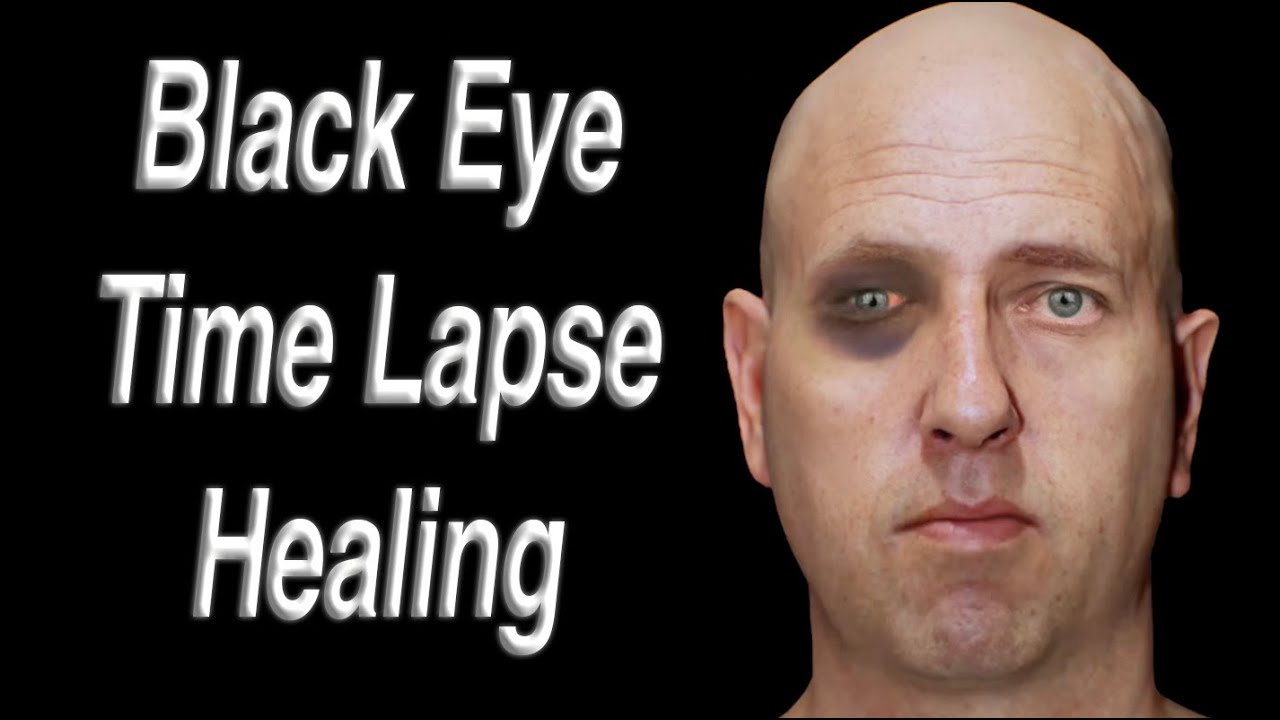This image appears to be a thumbnail for a YouTube video, featuring a meticulously photoshopped photograph of a bald Caucasian man, likely in his late 30s to mid-40s. The man faces the camera directly, showcasing a prominently blackened right eye, which may appear artificial and computer-generated. His face, clean-shaven and devoid of any notable features except for light pale green eyes and eyebrows, is set against a flat black background. On the left-hand side of the image, the white text with grey shading boldly reads: "Black Eye Time-Lapse Healing." The text is in a regular but embossed font style. This suggests that the video documents the man's healing process, possibly through a series of daily photos compiled into a sped-up sequence, highlighting the recovery of his black eye.